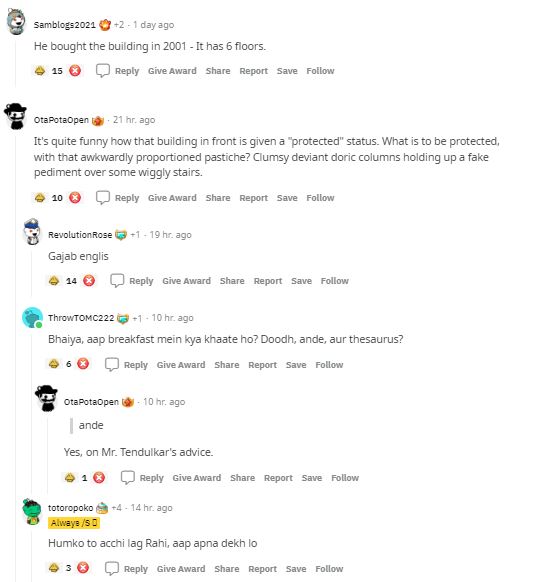**Screenshot Description:**

The screenshot captures a lively discussion on an unknown social network platform. The conversation revolves around a property related post by Sam Bloggs in 2021, where he mentions purchasing a six-floor building in 2001. Users seem to engage in a humorous debate about the architectural merit and historical preservation of a neighboring building, which they describe as awkwardly proportioned with clumsy Doric columns holding a fake pediment above wiggly stairs.

**Transcript of Key Comments:**

1. **Sam Bloggs (2021)**:
   - Context: Describes his purchase of a six-floor building in 2001.
   - Comment: "...It's quite funny how that building in front is given a protected status. What is to be protected with that awkwardly proportioned pasty, clumsy deviant Doric columns holding up a fake pediment over some wiggly stairs..."

2. **Revolution Rose**:
   - Comment: "Good job in glass, whatever that means..."

3. **Throw Tom C 222**:
   - Comment: "Budla at breakfast, Maine, Kaya, Nate, oh, dude, uh, Ante, or the Thorist."

4. **Otopata Open**: 
   - Comment: "On day, yes, on Mr. Tedulokar's advice."

5. **Toto Ro Poco**:
   - Comment: "Unco to Achilag, Rafi Apina Death Low."

The colorful array of user comments ranges from cryptic phrases to seemingly enthusiastic discussions about architectural details and preservation opinions.